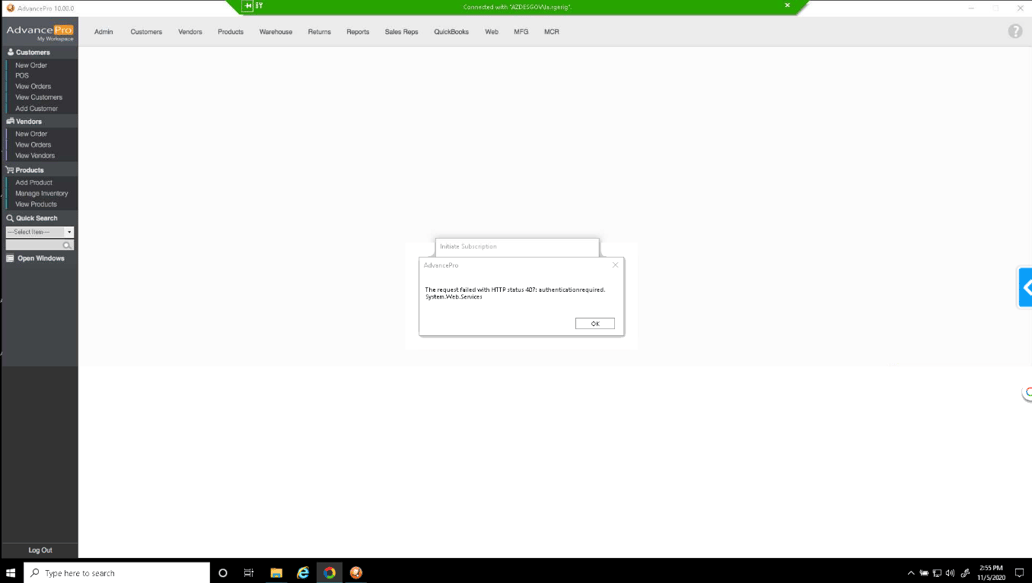In this online screenshot, the very top features a small green banner with white text. Along the entire left-hand side is a vertical gray banner, functioning as a library or menu. At the top of this gray banner, the word "Advanced" is displayed, with various information tabs listed below it.

Directly beneath this gray banner is a lighter gray horizontal banner with additional tabs that can be clicked, though their text is not easily readable.

Centrally, within the main body of the screenshot, there are a couple of pop-up windows. In the bottom-right corner of the first pop-up, a small button labeled "OK" can be seen.

Finally, at the very bottom of the screenshot, a black banner stretches across, showcasing the computer screen icons.